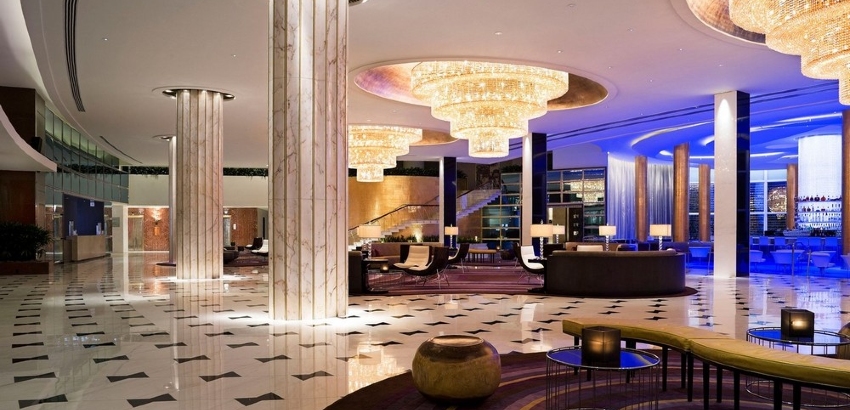The image captures the grandiose lobby of a ritzy hotel or resort, characterized by an expansive, rectangular space that is twice as wide as it is tall. The floor gleams with white marble tiles interspersed with black bowtie patterns, creating a striking and polished look. Dominating the scene are three enormous chandeliers descending from the high ceiling, designed like upside-down tiered wedding cakes and emitting a warm, golden glow akin to sunlight.

The lobby is anchored by two massive Ionic columns, subtly adorned without intricate flourishes, stretching impressively from floor to ceiling. These columns, likely made of marble, have vertical lines running through them, enhancing their grandeur. Towards the center of the room, a circular seating arrangement consists of brown, high-back chairs and plush sofas placed atop burgundy rugs, flanked by various end tables and lamps.

On the right side of the image, a bar area stands out, illuminated by a vivid blue light, with stools neatly arranged. Additionally, a staircase with a metal and wooden railing adds to the sophistication of the space. The back of the lobby features a separate room, bathed in a softer purple hue, and supported by brown pillars, extending the opulent atmosphere. Overall, this luxurious setting, with its attention to detail and elegant design elements, evokes a sense of high-end comfort and sophistication, suitable for hosting various upscale events.